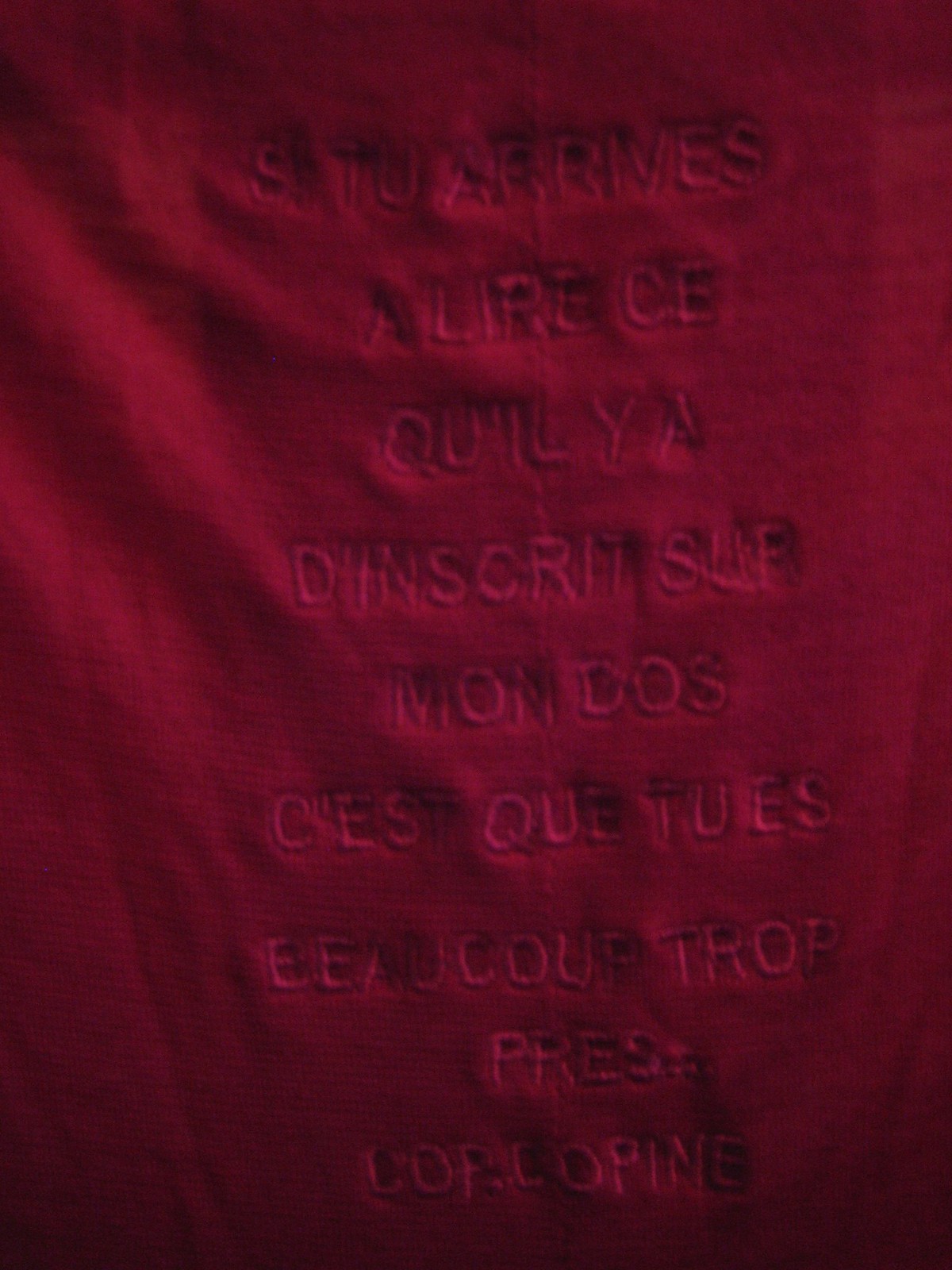This evocative photograph captures an intricate piece of fabric rendered in deep, textured reds that darken to near-black shadows toward the bottom. The fabric bears nine distinct rows of text, possibly in French or Latin, though the shadowy ambiance makes it challenging to decipher the exact script or language. Each line of text is composed of one to three words, meticulously either pressed into or embroidered upon the material in a color strikingly similar to the fabric itself. The subtle motion and folds in the fabric create an interplay of light and shadows, adding a sense of depth and mystery to the image.